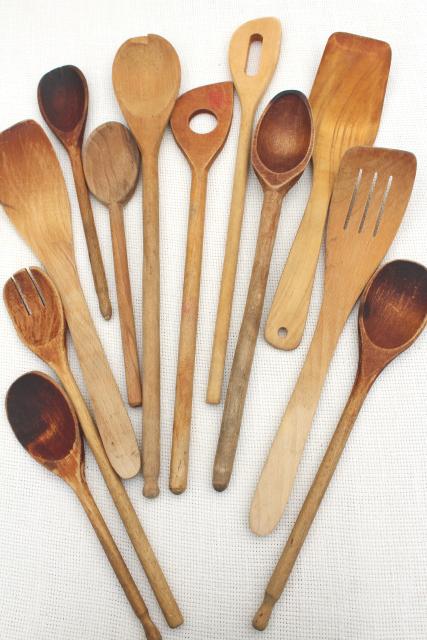This photograph showcases a top-down view of a variety of wooden kitchen utensils arranged in a half-circle on a white, linen-like textured background. The utensils include an assortment of wooden spoons, spatulas, and a unique spork-like utensil. Some spatulas feature distinctive cutouts, such as slits, a large circular hole, and an oval hole. The wood varies in color from a dark brown, possibly due to extensive use or a darker type of wood, to a lighter brown, indicative of different wood types or less wear. Notably, two spoons positioned at the edges of the half-circle are darker, whereas the spatulas tend to be lighter. The arrangement and variety provide a rich visual detail of these well-crafted wooden kitchen tools.